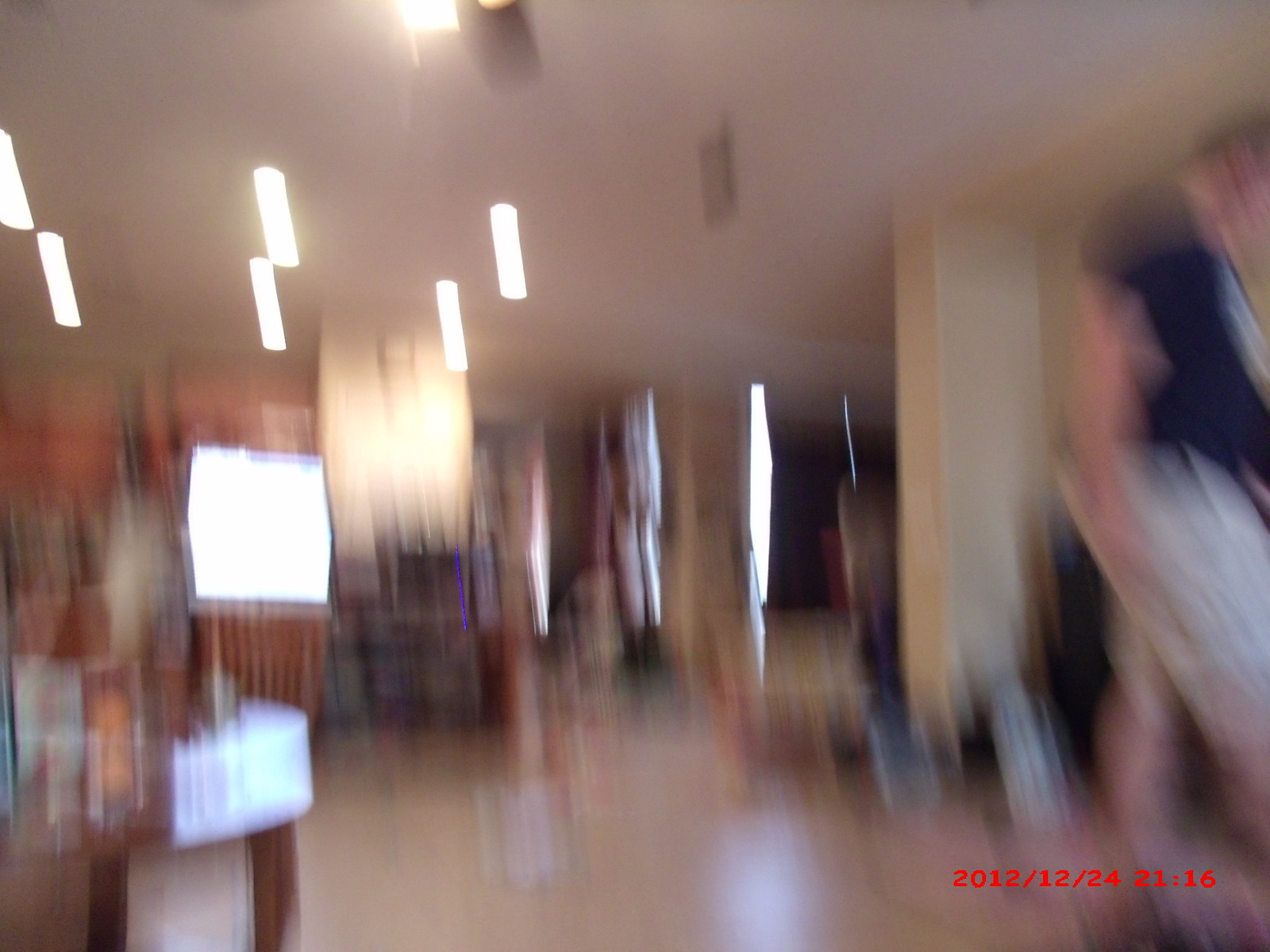The image is extremely blurry, giving the impression of the room spinning. In the lower right-hand corner, red text indicates the date and time: 2012/12/24, 21:16, suggesting it is Christmas Eve at around 9:16 PM. On the right side of the image, we can discern the side silhouette of a person. They appear to be wearing a dark-colored top, possibly navy blue or black, that exposes part of their arm, along with light-colored pants or khaki shorts. The room features several bright, white pendant lights hanging from the ceiling, creating double, ghost-like images due to the blur. The background includes a mix of neutral tones, with glimpses of what appears to be brown tables, brown curtains, and a reflective glass surface suggesting a potential setting of a restaurant, cafe, or lobby. There is also a notable large yellow column on the right side of the photo.